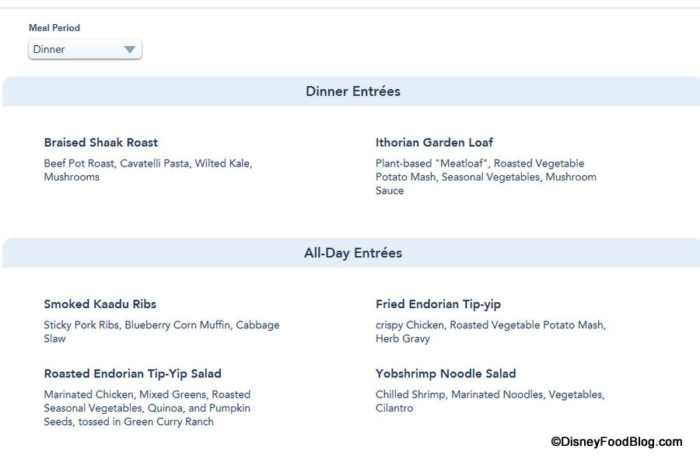The screenshot displays a section of the DisneyFoodBlog.com website, specifically highlighting meal options under the "Dinner" category. At the top, the page indicates the meal period with a label that reads "Dinner" and a drop-down arrow suggesting more menu options. Below this, there is a gray, narrow box titled "Dinner Entrees" in black lettering, listing menu items such as "Braised Shank Roast" and "Ethorian Gordon Loaf."

Further down, another small rectangular box labeled "All Day Entrees" in black text details additional options. On the left side, it lists "Smoked Kadu Ribs" and "Roasted Endorian Tip-Yip Salad," while the right side includes "Fried Endorian Tip-Yip" and "Yob Shrimp Noodle Salad." At the bottom of the image, the website’s copyright, DisneyFoodBlog.com, is noted, indicating that the menu is affiliated with Disney, likely from one of their properties such as a cruise or theme park attraction like Disney World.